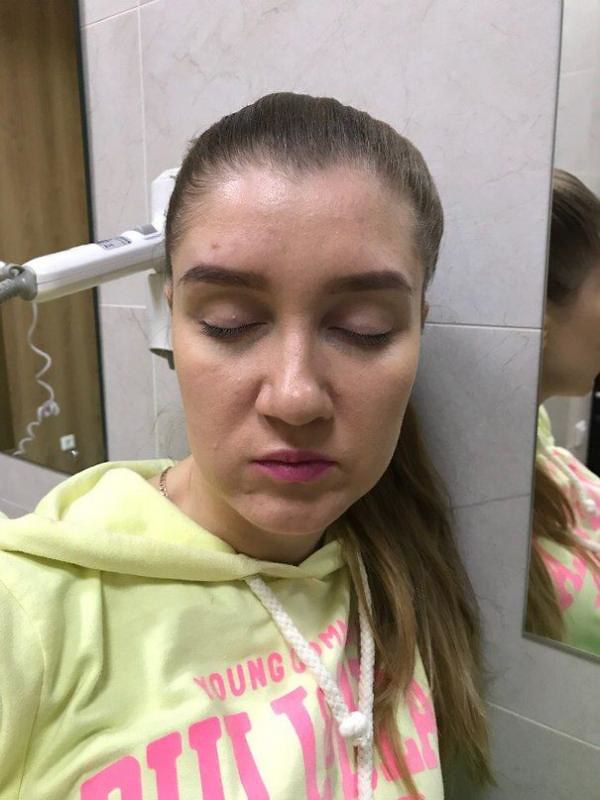This color photograph is a close-up of a young Caucasian woman who appears to be in a bathroom, leaning against a wall adorned with one-foot square white tiles. Her long, dark blonde hair is pulled back into a ponytail that gracefully falls over her left shoulder, revealing her closed eyes accentuated with purplish eyeshadow and pink lipstick. She is wearing a pale yellow hoodie featuring pink text on the front, partially visible in the shot that extends from the top of her head to her chest. On either side of her head are two rectangular mirrors, reinforcing the bathroom setting, further emphasized by the visible hairdryer mounted on the wall with its handle sticking out and its cord hanging down. Additionally, a light switch and an electrical cord can be seen in the background. The reflective surfaces and the faint gold necklace she wears add subtle details to this serene composition.